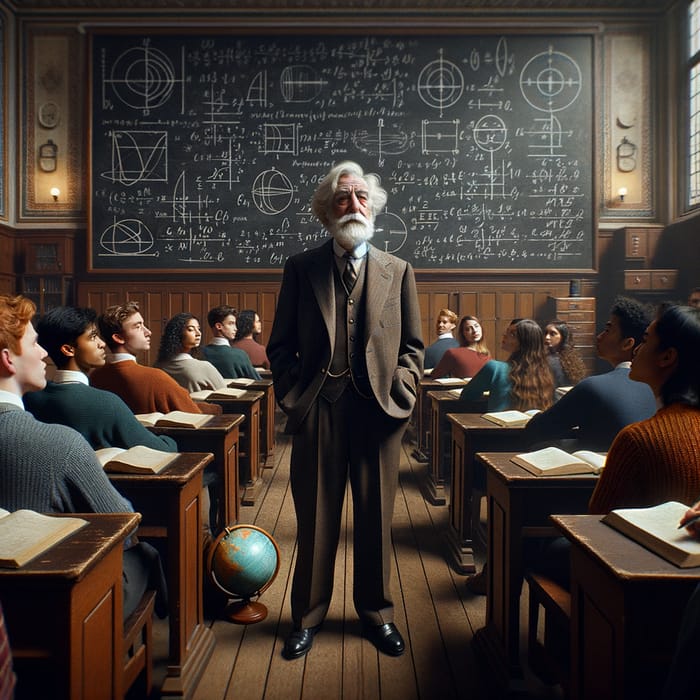The hyper-realistic painting portrays an advanced physics classroom filled with an array of intricate details. In the center stands an elderly professor, an intellectual figure marked by his white hair and full beard. He dons a formal, three-piece brown suit, complete with a brown tie against a crisp white shirt, and wears polished black shoes. His hands rest in his pockets as he stands thoughtfully next to a light teal globe that sits on the wooden floor. The classroom itself is populated by students seated in neat, orderly rows of wooden desks. These students, enraptured by the professor's presence, are dressed in colorful vests and sweaters—shades of orange, gray, green, and blue.

The front of the classroom features a large chalkboard, towering high with a plethora of mathematical formulas, equations, and scientific diagrams meticulously drawn in chalk. The walls are lined with wooden paneling and decorated with various hanging items, while sconces cast warm light across the room. Windows on the right-hand side allow natural light to filter in, complementing the characteristically academic ambiance. Despite the overall realistic depiction, subtle oddities hint at an AI-generated origin, such as a female student whose head appears unusually turned, and the blackboard positioned implausibly high above reach.